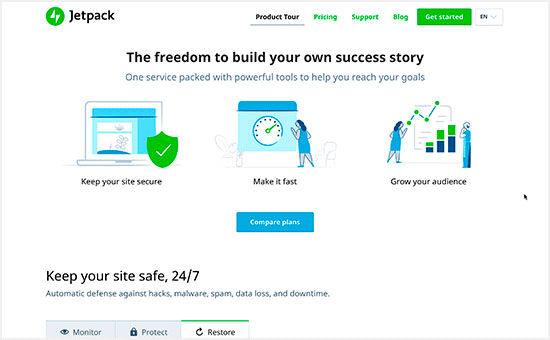The image depicts the homepage of the "Jetpack" website, featuring a streamlined and user-friendly layout. At the top left, the Jetpack logo is prominently displayed, identifiable by a green symbol. Along the same line to the right, the navigation menu includes options for "Product Tour," "Pricing," "Support," "Blog," and "Get Started." A language selection tab is situated on the far right of the navigation bar.

Beneath the navigation bar, a bold headline proclaims, "The Freedom to Build Your Own Success Story," underscored by a tagline that describes Jetpack's services: "Our service packed with powerful tools to help you reach your goals, keep your site secure, make it fast, and grow your audience."

Further down, there's a call-to-action button inviting viewers to "Compare Plans," followed by detailed sections elaborating on the security features Jetpack offers. These sections highlight the service's automatic defenses against hacks, malware, spam, data loss, and downtime with bullet points stating, "Keep Your Site Safe," and "Monitor, Protect, and Restore."

The image suggests that Jetpack is a comprehensive website hosting and management service, emphasizing the importance of site security, performance optimization, and audience growth. The visible portion of the page provides a concise but detailed overview of Jetpack's key offerings, targeting prospective users looking to enhance and protect their websites.